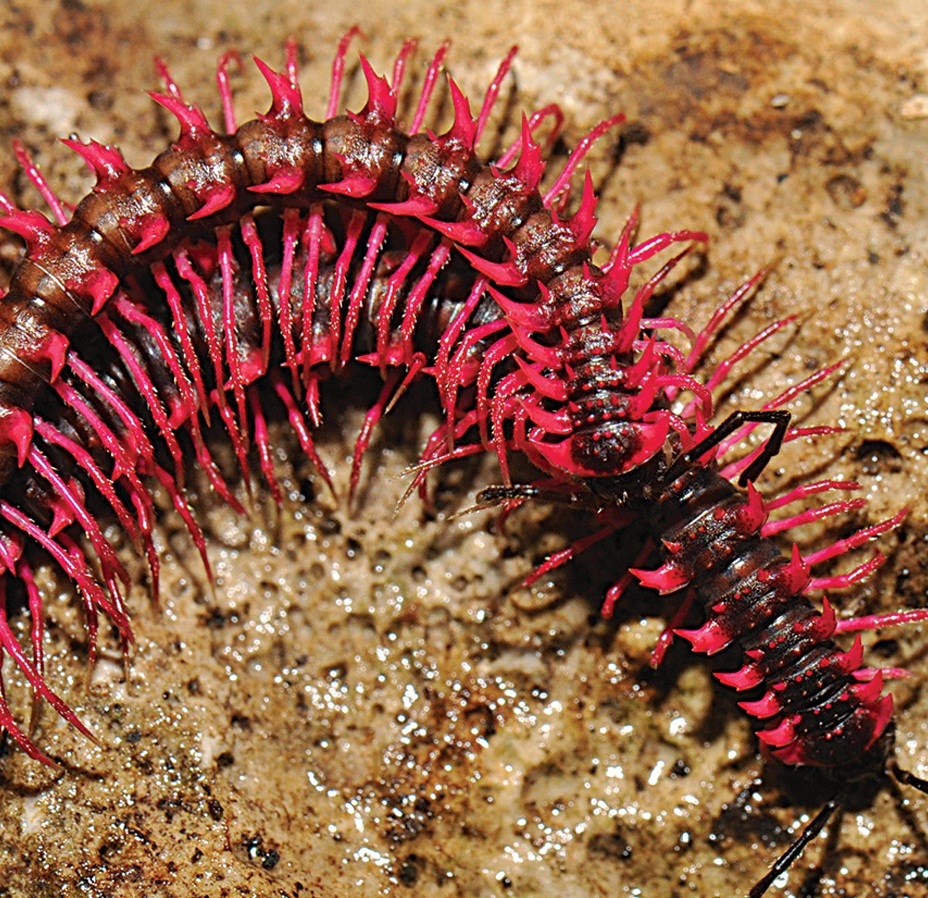In this detailed macro photograph, two exotic-looking centipedes are captured in exquisite detail, each boasting dark-bodied exteriors with vibrant red legs and defensive red protrusions on each segment. The insects are positioned in a huddled manner, with one seemingly on top of the other, forming what resembles an upside-down "U" shape. Their antennas rest in a relaxed position, emphasizing a tranquil moment. The backdrop reveals a moist, grainy surface, likely dirt or sand, intermixed with darker bits and reflective patches, hinting at a recently dampened environment. The centipede on the bottom is dark brown with striking red spikes and legs, while the upper one appears slightly lighter in brown coloration, but similarly adorned with vivid red legs and spike-like protrusions. The 8-inch by 8-inch image vividly contrasts the centipedes' vibrant colors against the light brown, muddy terrain they inhabit, highlighting the intricate texture and natural setting of these fascinating creatures.